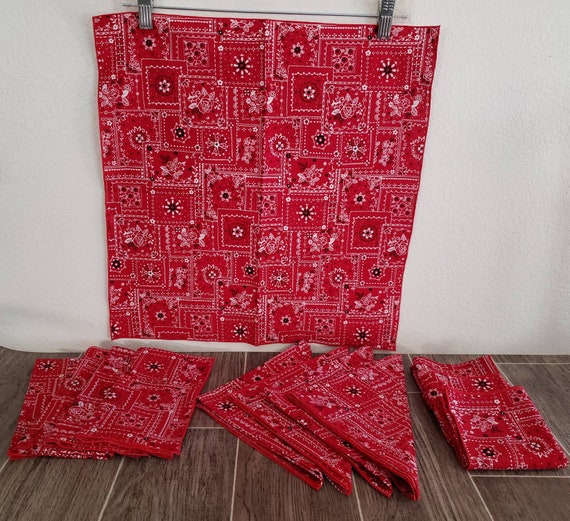The image shows a detailed display of red patterned fabric with a back wall and floor as a backdrop. The fabric has a vibrant red color, featuring white-outlined squares each adorned with intricate black and white floral designs and circular patterns. The main piece of fabric is hung on a white wall using a hanger and two metal clips, clearly showcasing its detailed pattern. The floor, consisting of medium and dark brown hardwood sections with light gray grout lines, complements the display. On the floor, multiple pieces of the same fabric are arranged: to the left, four rectangularly folded pieces overlap; in the middle, three more lie stacked in rectangles; to the right, several pieces are folded into squares. Though the fabric's use is unspecified, it might serve as tablecloths or bandanas, given its versatile presentation. There is no text in the image to further explain the items.